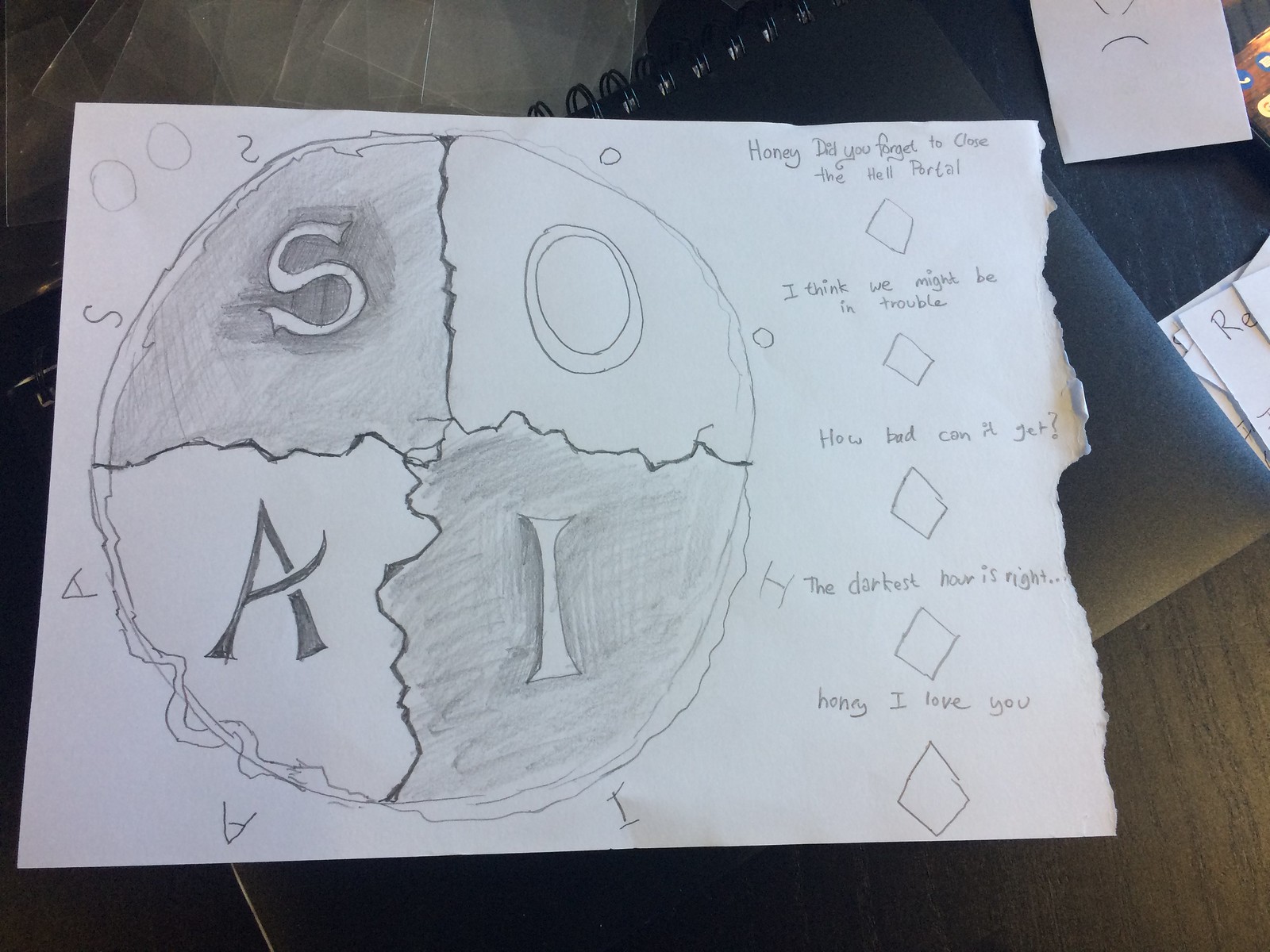A detailed caption for the image could be:

"A detailed pencil drawing on a piece of paper rests atop a black booklet, which itself is placed on a wooden table. To the right of the booklet, additional sheets of white paper are visible. The drawing features a large circle surrounded by various letters and text. On the left side of the circle, the letters 'O' and 'I' are vertically aligned, while 'S' and 'A' are positioned to the left. Encircling the top and right side of the circle are the letters 'I-A-A-S-S.'

To the right of the circle, a conversation is depicted in a series of diamond-shaped text bubbles:
- 'Honey, did you forget to close the hell portal?'
- 'I think we might be in trouble.'
- 'How bad can it get?'
- 'The darkest hour is right.'
- 'Honey, I love you.'

The entire composition suggests a humorous and possibly ominous scenario, rendered with simple yet effective pencil strokes."